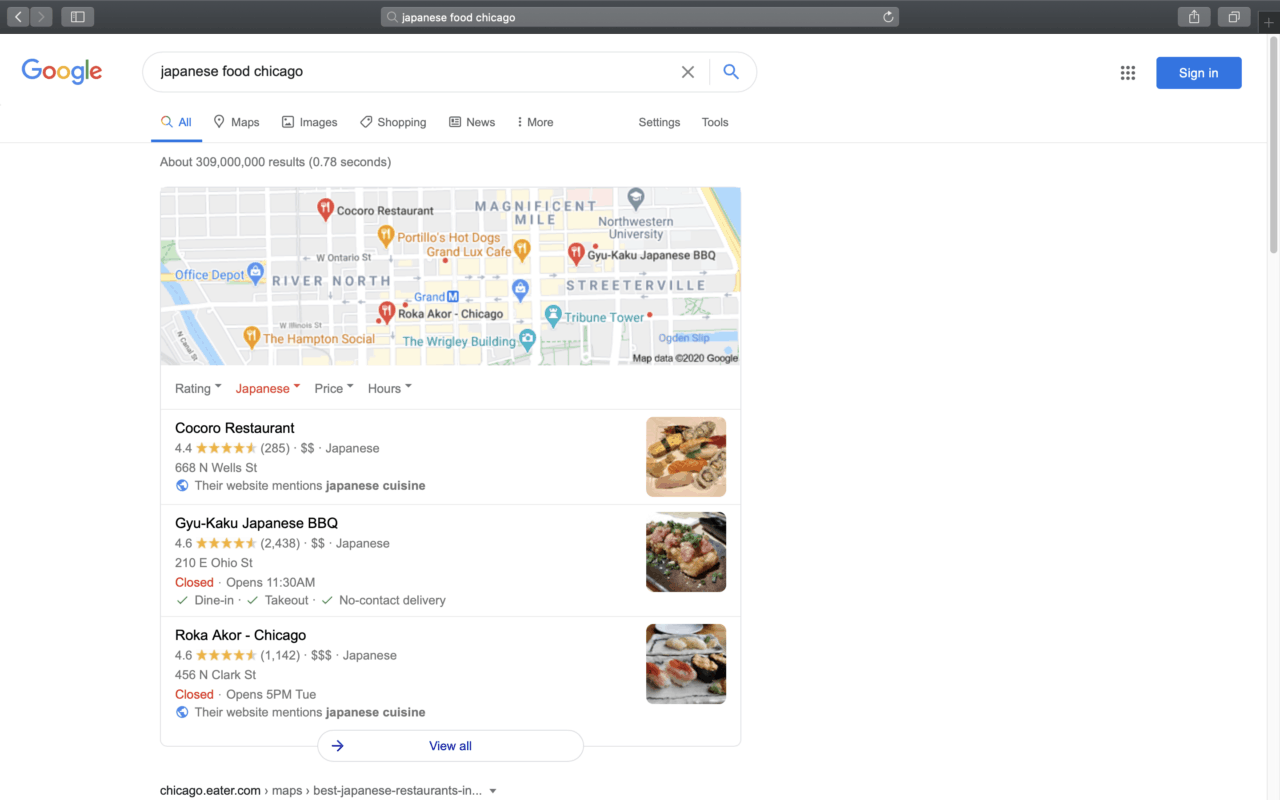A Google search result page is displayed with a search bar at the top, featuring a thin black border and the query "Japanese food Chicago." Below the search bar, the classic Google logo appears on the left, with a blue "Sign in" button on the right. Directly beneath this bar are navigational tabs labeled "All," "Maps," "Images," "Shopping," "News," "More," and tools options. The main portion of the screen displays a Google Maps snapshot focused on the Magnificent Mile in Chicago, pinpointing various locations with red markers. Three Japanese restaurants are listed beneath the map: Kokoro Restaurant, Gyu-Kaku Japanese BBQ, and Roka Akor Chicago.